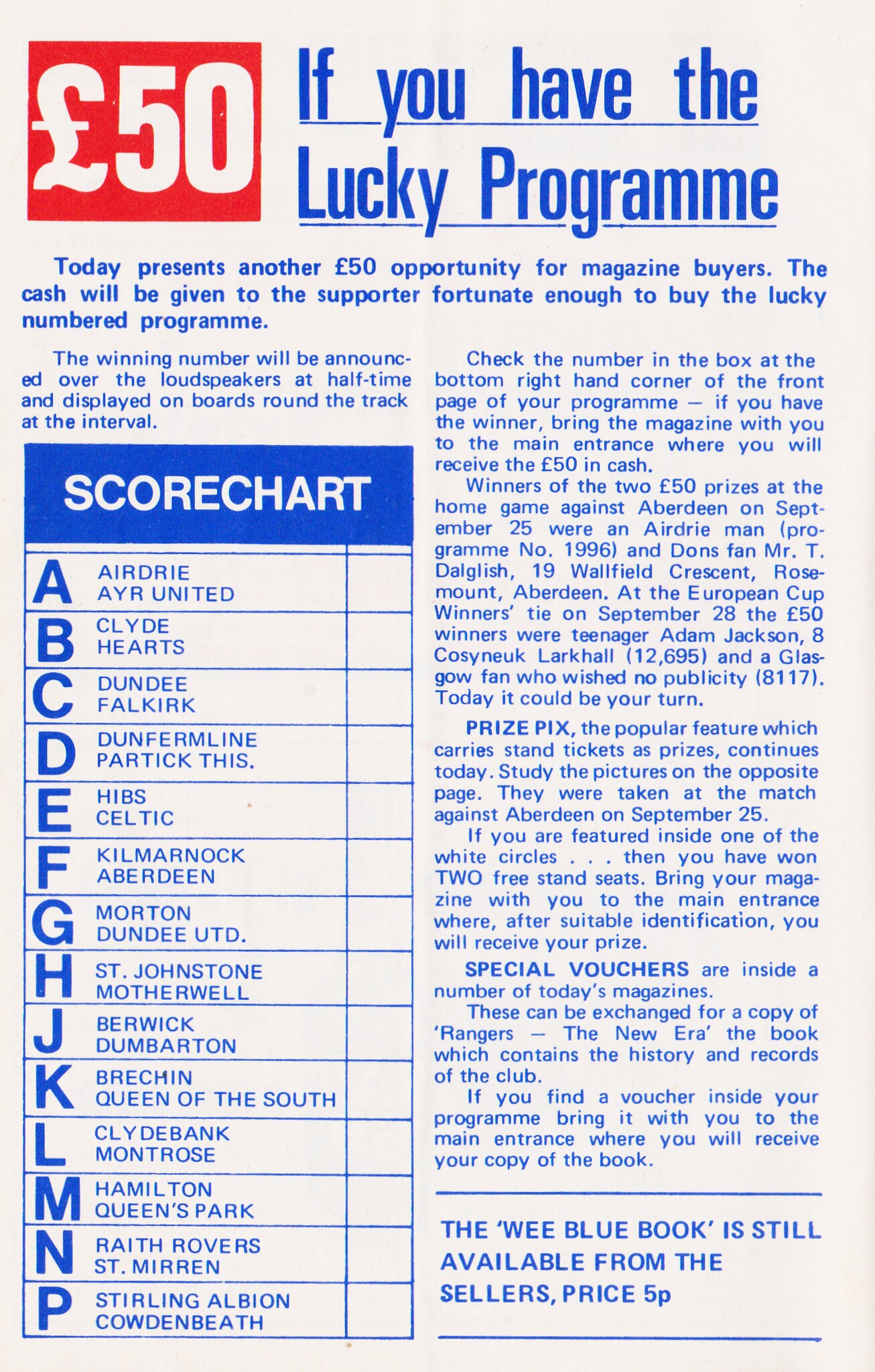The image is a detailed advertisement taken from a magazine page. It announces a contest titled, "If You Have the Lucky Program," with a subtitle beneath it stating, "Today presents another 50-pound opportunity for magazine buyers." To the left of this title is a prominently displayed red square containing the amount "50 pounds" in white text. This signifies the cash prize to be given to the supporter fortunate enough to buy the lucky numbered program.

The page is neatly divided into several sections. On the right side, the column is filled with explanatory text about the contest. On the left, there is a section that includes a score chart titled "Scorecard," which lists a series of teams or places from A to P in an alphabetically ordered format. For example, 'A' stands for Ayr United, 'B' for Clyde Hearts, and 'P' for Stirling Albion Cowdenbeath. Additionally, it mentions that "The wee blue book is still available from sellers, priced at 50 p.m." This comprehensive arrangement of sections and detailed information creates a clear and attractive layout for the readers.